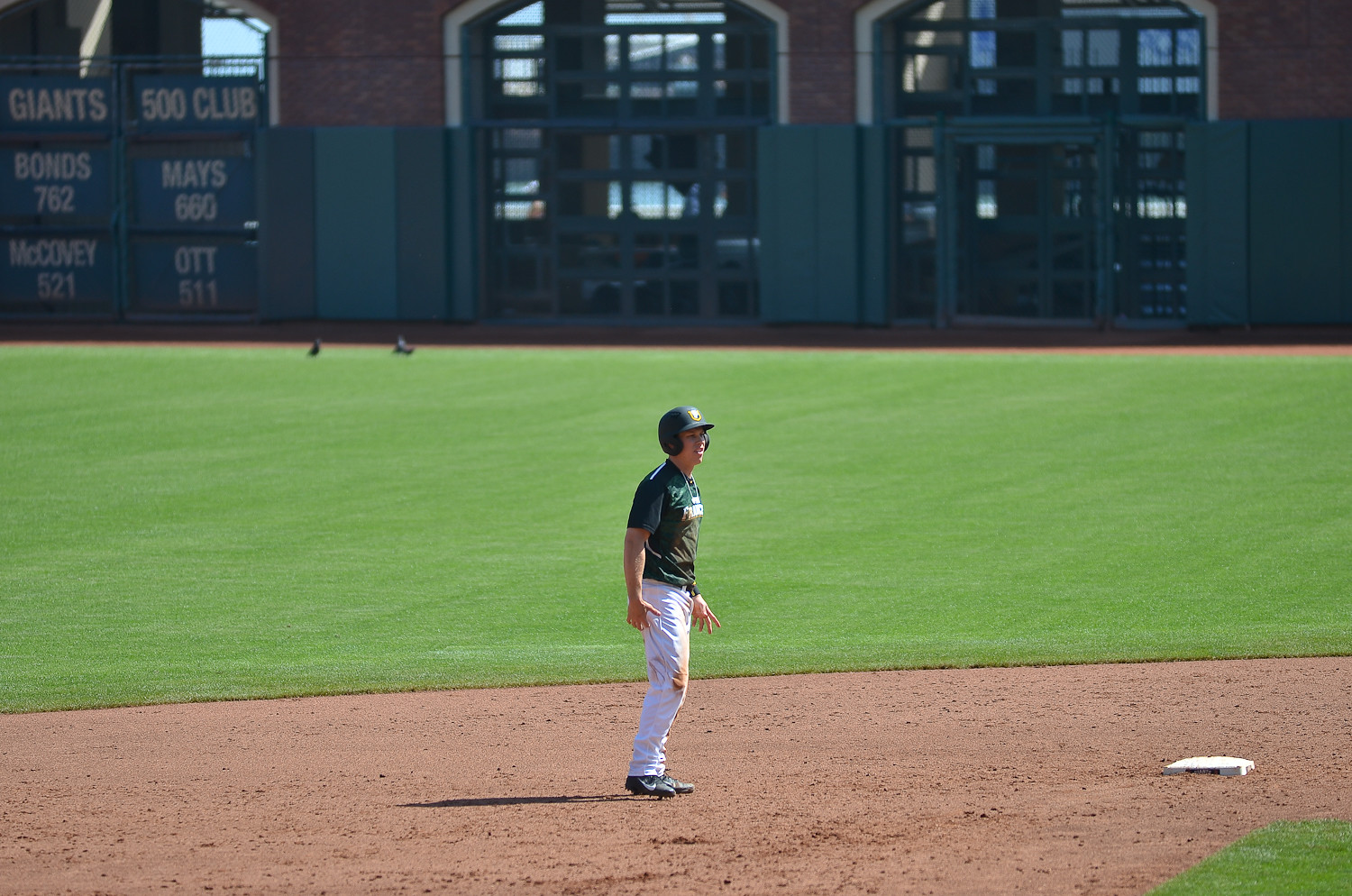This full-color photograph captures the intensity of a baseball game on a bright, sunny day. A single runner, dressed in a green helmet, green jersey with white and yellow trim, and scuffed white pants, stands leading off from second base. The dirt stains on his knee and jersey suggest he has already made a daring slide. He is positioned right at the center of the field, bathed in sunlight, casting a shadow behind him. His green Nike cleats dig into the well-maintained grass as he attentively watches the action at home plate. The surroundings suggest a professional baseball park, with green padding on the distant wall and historical Giants milestones proudly displayed: Bonds 762, Mays 660, Ott 511, along with others that are partially obscured. Birds are seen landing out in the outfield near the warning track, adding a touch of life to this vivid sports scene.